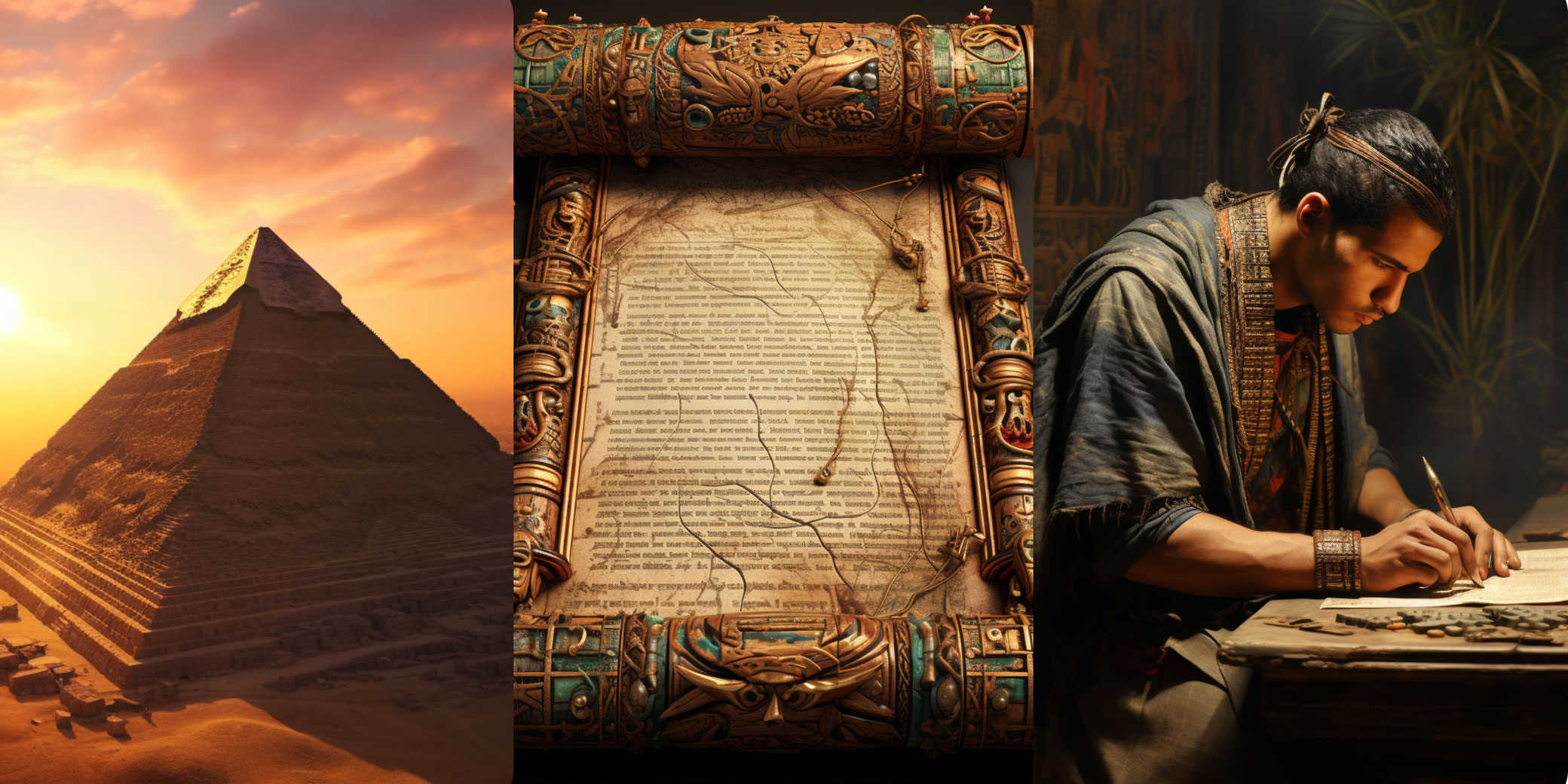The image is a high-quality digital art collage featuring three evenly sized panels. On the far left, the first panel showcases the majestic Great Pyramid of Giza at sunset. The pyramid displays a partially restored base with weathered, cracked siding in the middle, leading up to a golden capstone that glistens in the sun's warm light. The sky above is painted in a gradient of pastel pinks, purples, and a hint of gray clouds, adding to the serene yet grand atmosphere.

The center panel highlights an ancient scroll encased in an exceedingly ornate frame. The scroll itself appears aged and weathered, with illegible text. The elaborate frame surrounding the scroll is intricately detailed, possibly crafted from green jade with bronze or copper carvings, or wood painted green. It is adorned with exquisite designs, showcasing impeccable craftsmanship without depicting specific images.

The far-right panel depicts a man dressed in traditional clothing, seemingly from ancient Asian culture. He is seated at a table, engrossed in writing on a sheet of paper. His attire includes dark blue, poncho-like garments with lighter-colored, striped fabric draped around his neck. He sports a band tied around his black hair, and his dark brown skin hints at his cultural background. Behind him, you can spot plants and a painting, adding depth and context to the setting of the scribe diligently at work.